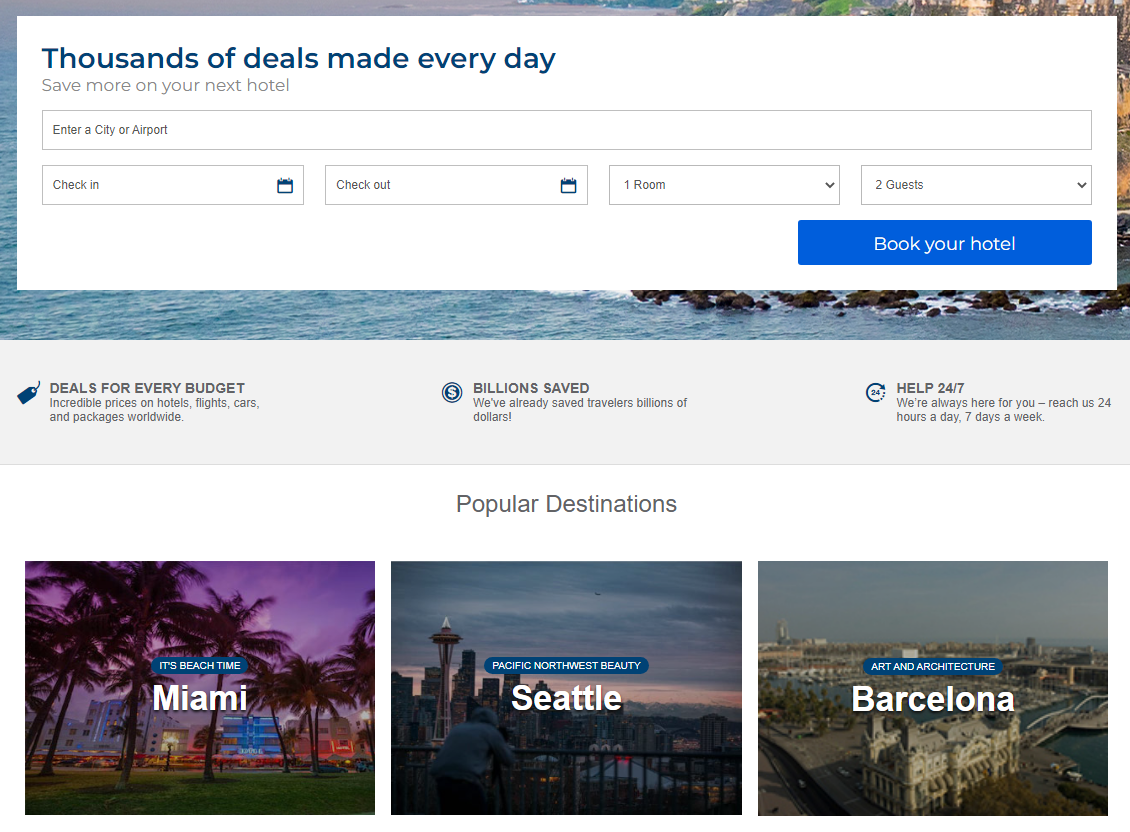The screenshot captures a promotional banner from a travel deals website. Dominating the top portion, a large white box spans almost the entire width, prominently featuring the text “Thousands of deals made every day” in bold lettering. This box contrasts sharply with the background, a serene ocean view subtly visible around the edges, showcasing a rugged shoreline with rocky hills.

Directly above this white section, nestled in the top navigation area, is a smaller message reiterating "Thousands of deals made every day." Below the main slogan within the white box, a secondary line of text encourages users to "Save more on your next hotel."

The central area of the banner includes a user-friendly search interface. This comprises an input field labeled "Enter a city or airport," followed by selection boxes for "Check-in," "Check-out," "One room," and "Number of guests." To the right of these input fields, a prominent button urges users to "Book your hotel."

Beneath the white box, a gray section offers additional value propositions with the phrases: “Deals for every budget,” “Billions saved,” and “Help 24/7.” Finally, the banner concludes with a section dedicated to "Popular Destinations," showcasing a variety of travel options.